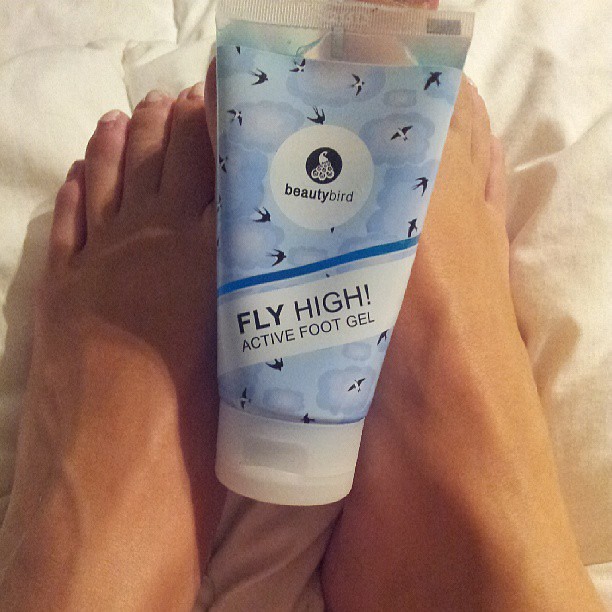The image features a close-up of a woman's feet, angled with the toes pointing towards the top of the picture and the ankles at the bottom. Her feet rest on a white bedding towel, and they cradle a bottle of Fly High Active Foot Gel by Beauty Bird. The bottle, adorned with blue-gray clouds and bird designs, has a white cap pointing downwards. The photo, likely an advertisement, contains no text other than the product label and showcases a serene indoor setting, emphasizing both the foot gel and the comfort it aims to provide. The colors in the image include light blue, dark blue, black, cream, off-white, and tan, contributing to a calm and soothing aesthetic.